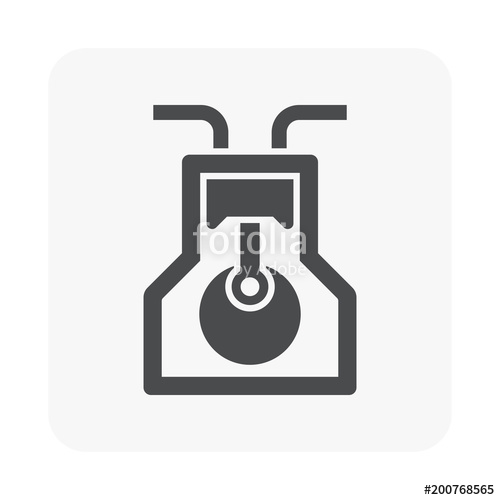This black and white line art illustration, centered in a square format with a light gray background, prominently features a complex icon resembling a beaker. The beaker is outlined with a heavy black line, narrow at the top and broadening towards the base with tapered sides. Inside the beaker, there is a black circle on a white background near the bottom, topped by a smaller white circle and an upward-facing rectangle. Extending from the neck of the beaker are two straws or pipes, pointing outward to the left and right. Overlaying the image is a watermark reading "Fotolia by Adobe" in light white text. In the bottom right corner, a serial number "#200768565" is displayed in black text. The illustration's style is reminiscent of stock images or clipart.